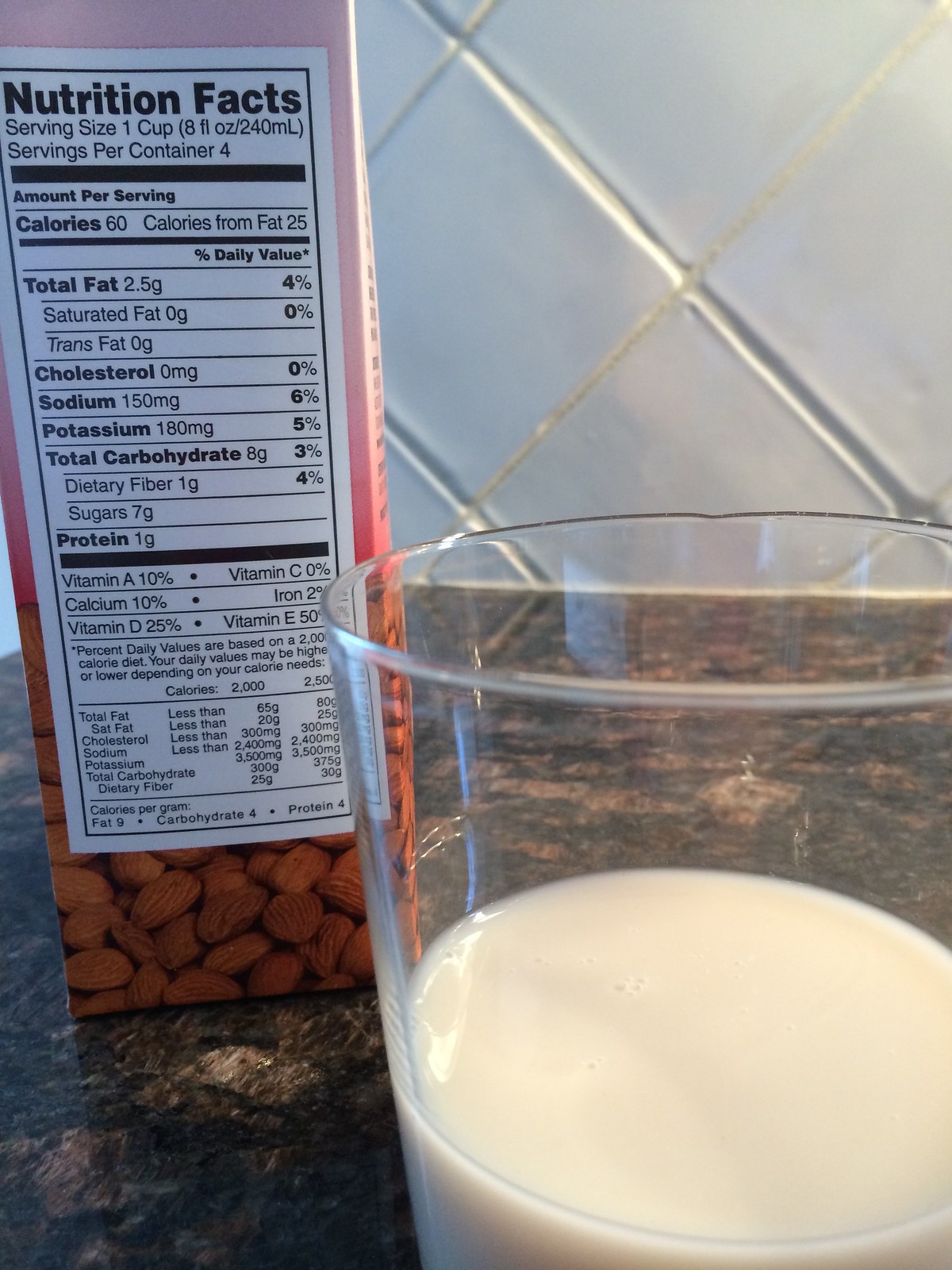This image features a carton that likely contains almond milk. The prominent side of the carton, visible in the picture, displays the nutrition facts which are positioned on the left side, extending from the bottom right up to the top center of the carton. The majority of the image is centered around a glass filled with a white liquid, presumably the almond milk from the carton, placed on a countertop. Positioned at the bottom part of the carton are illustrations or photographs of whole almonds, emphasizing the contents. The nutrition facts indicate that a serving size is 1 cup (8 fluid ounces).